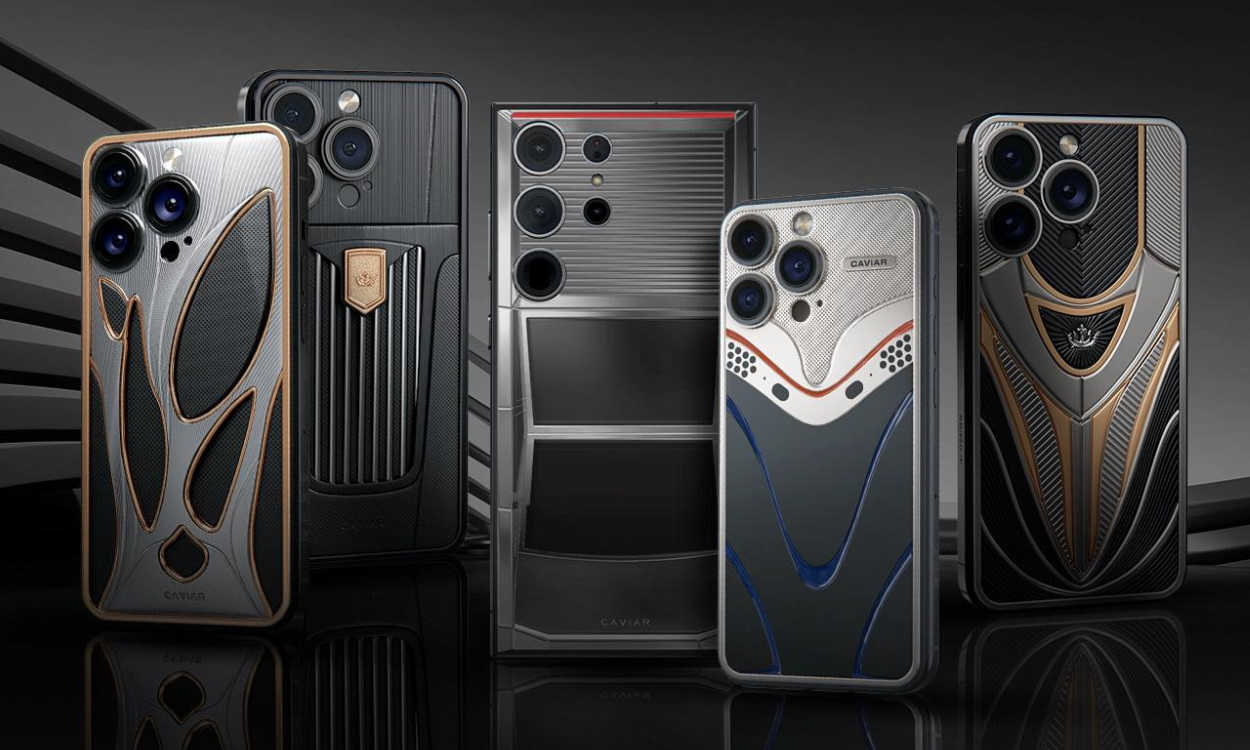This image showcases the backs of five distinct smartphones, all positioned against a sleek, shiny black table that reflects the devices, with a matching black background. 

- **First Phone (Left)**: This device features a distinctive black and silver case with leafy-shaped patterns, trimmed in gold. It also houses three camera lenses positioned in the top left corner.
  
- **Second Phone**: This smartphone is encased in a black rubberized cover with three camera lenses on the left side. It features a prominent gold emblem resembling a shield or crown in the center, accentuated by silver stripes.
  
- **Third Phone**: With a sleek silver and black exterior, this phone stands out with its three vertically-aligned camera lenses on the left and two additional smaller lenses to the right.
  
- **Fourth Phone**: Slightly shorter than its counterparts, this device has a top half in silver and a bottom half in black, with a striking red trim separating the two areas. A blue decoration adorns the center, and the entire phone is bordered in silver.
  
- **Fifth Phone (Right)**: This final smartphone showcases a mix of black, gold, and silver elements. It includes three camera lenses on the left side, a silver-trimmed black area that could resemble a speaker, and the word "caviar" inscribed at the bottom.

Overall, each phone displays a unique and intricate design, ranging from leafy patterns to emblematic shields and sleek metallic finishes.